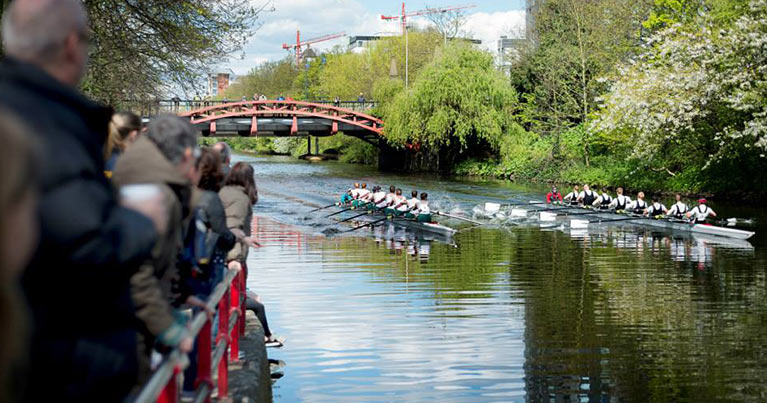The photograph captures a vibrant rowing race on a sunlit river framed by lush green trees. In the background, an orange copper-colored arched bridge crosses over the river, where several onlookers stand, gazing down at the rowers. The rowboats, long and narrow, each carry eight male rowers, their bodies aligned in single file, moving in synchronized unison. Their large oars slice through the water, propelling the boats backwards as they race towards the foreground. In the out-of-focus foreground, about ten spectators lean over a railing, their heads turned toward the race, eagerly watching the competition unfold. The scene is bustling with onlookers on either side of the water, all clad in puffer jackets, suggesting a crisp yet sunny day under clear blue skies.